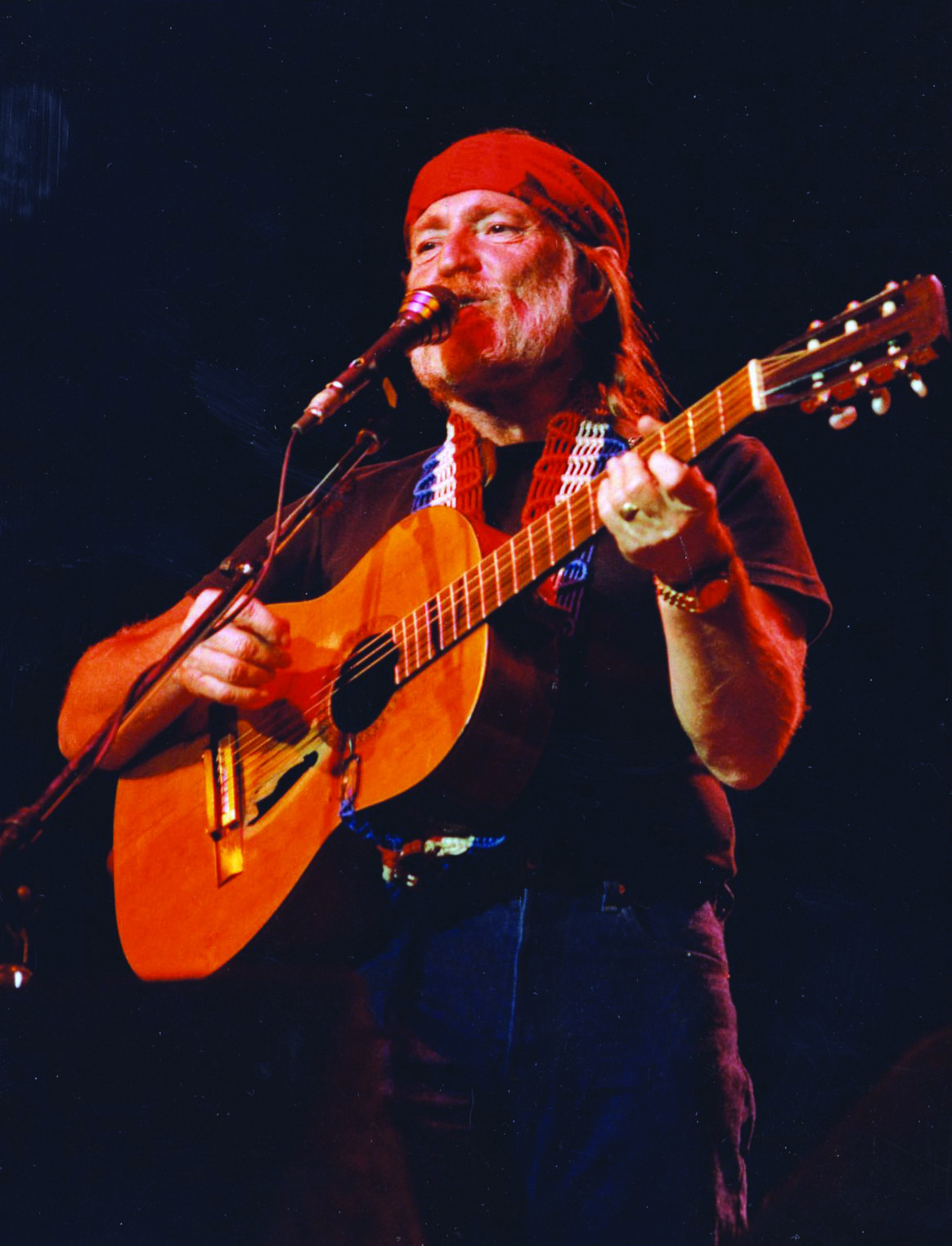This detailed photograph captures the legendary country singer Willie Nelson in the midst of a powerful performance on stage. He stands out vividly against the pitch-black background, creating an intimate spotlight effect. He is deeply engaged with his music, strumming a light brown wooden acoustic guitar, which features white pegs. The guitar is secured with a strap adorned in red, white, and blue stripes. Nelson is impeccably dressed in a short-sleeved black t-shirt, dark blue jeans, and a black belt, accessorized with a gold watch on his left wrist and a gold ring on his ring finger. His head is crowned with a red bandana wrapped around his hair, and his white beard is visible as he sings into a silver microphone mounted on a stand. The black flexible wire of the microphone is wrapped around the stand, further focusing the viewer's attention on Nelson's passionate performance. His gaze is directed towards the crowd, capturing the essence of his connection with his audience.